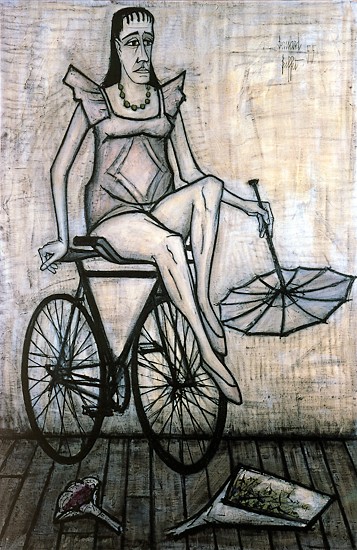The image portrays a melancholic woman perched precariously on the handlebars of a bicycle, almost in a circus-like pose with her feet resting on the front tire. She clutches the seat of the bicycle with her right hand for balance, while her left hand holds an inverted parasol, its handle pointing upwards and its canopy facing downwards. Her elongated face, marked by a sad grimace, gives her a strikingly somber appearance. She is dressed in a top resembling a ballerina's leotard with flared shoulders, finishing just below her waist, and she wears a beaded necklace. Her long hair, with bangs framing her face, cascades down her back. The background features a wall with hues of brown, orange, and white, and a dark gray and brown wooden floor beneath the bicycle. On the ground in front of the bicycle lies what appears to be two bouquets of flowers, adding a touch of fragile beauty to the scene. The entire composition is rendered mostly in black ink with subtle tints of brownish-orange, giving it a monochromatic, sketch-like quality.